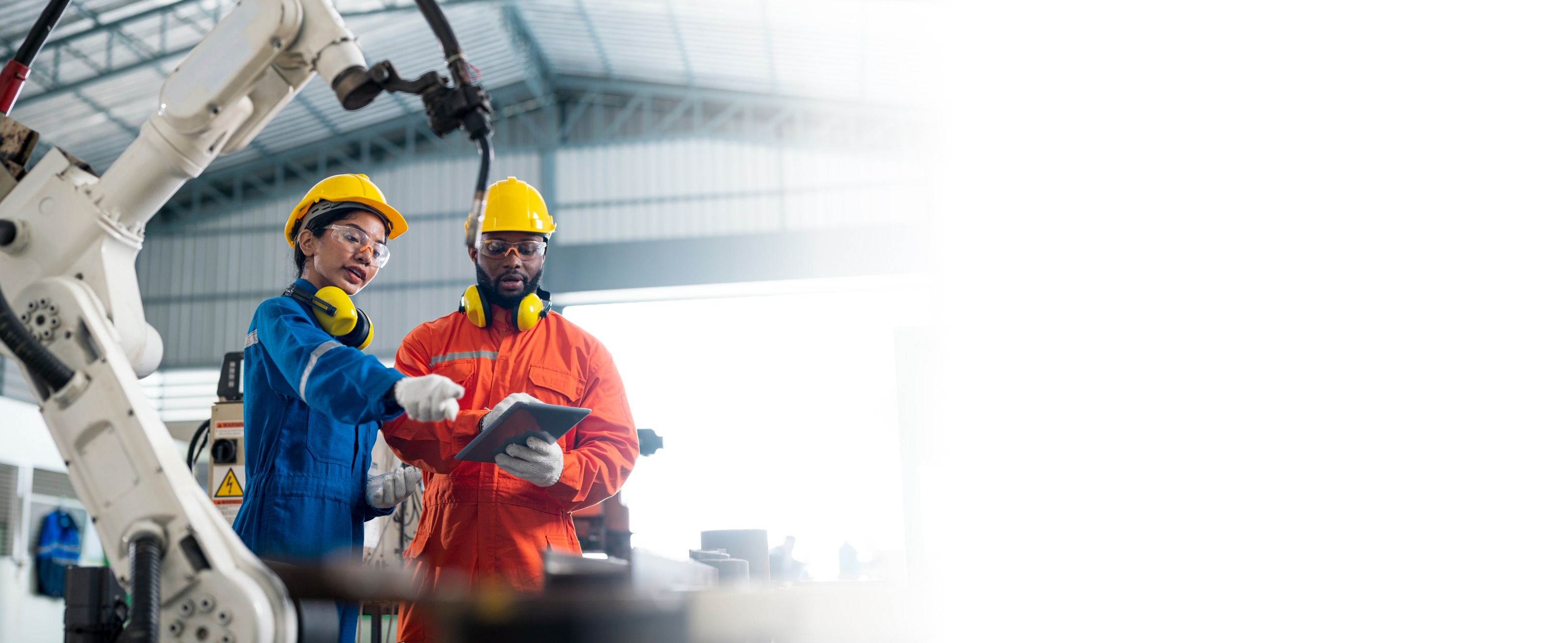In this detailed image, taken inside a vast warehouse or factory with metal roofing and a high ceiling, the scene is partially obscured by bright light streaming in from an open garage door on the right side, causing a glare that fades into whiteness. The setting reveals an industrial environment equipped with various robotic machinery, including a prominent robotic arm. 

In the foreground, a woman and a man are engaged in a task beside the machinery. The woman, wearing a green jumpsuit with reflective strips, a yellow helmet, clear goggles, and yellow earmuffs, and white gloves, is pointing at a gray tablet held by the man next to her. The man is dressed in an orange jumpsuit with white gloves, yellow earmuffs, and a yellow hat. Both individuals exhibit focused attention on the tablet, possibly discussing details related to their work. The mention of their ethnicities, an Asian young woman and a black young man, adds to the diversity represented in the image. Surrounding them are indications of advanced robotic technology, suggesting a modern, high-tech manufacturing or industrial process.